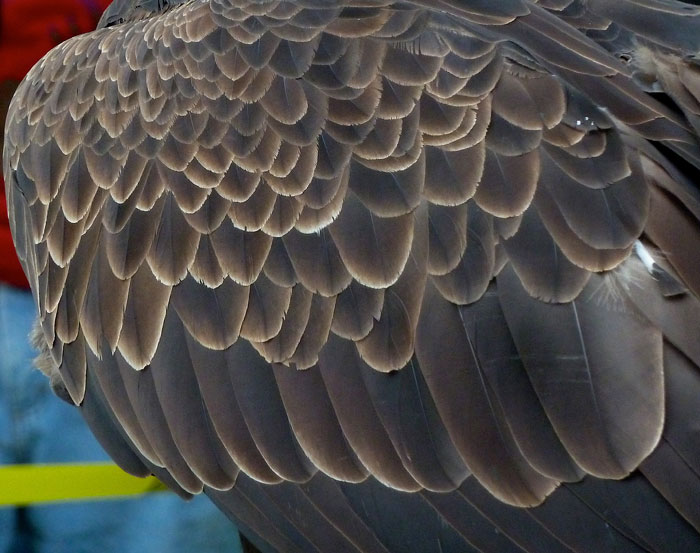This full-color, square photograph, likely taken indoors by a professional, offers an intimate close-up of a bird's wing, possibly a hawk or owl. The meticulously aligned brown feathers vary in size and texture, from light to dark shades, with some gold tinges at their ends. Light catches the edges, creating a subtle highlight. In the extreme lower left, a yellow bar intersects the image, while the background displays blue in the bottom left and red in the upper left corner. A partial view of the bird's head and the corner of its eye is visible in the upper left, emphasizing the bird's dense, layered plumage—an awe-inspiring testament to nature's intricate design.